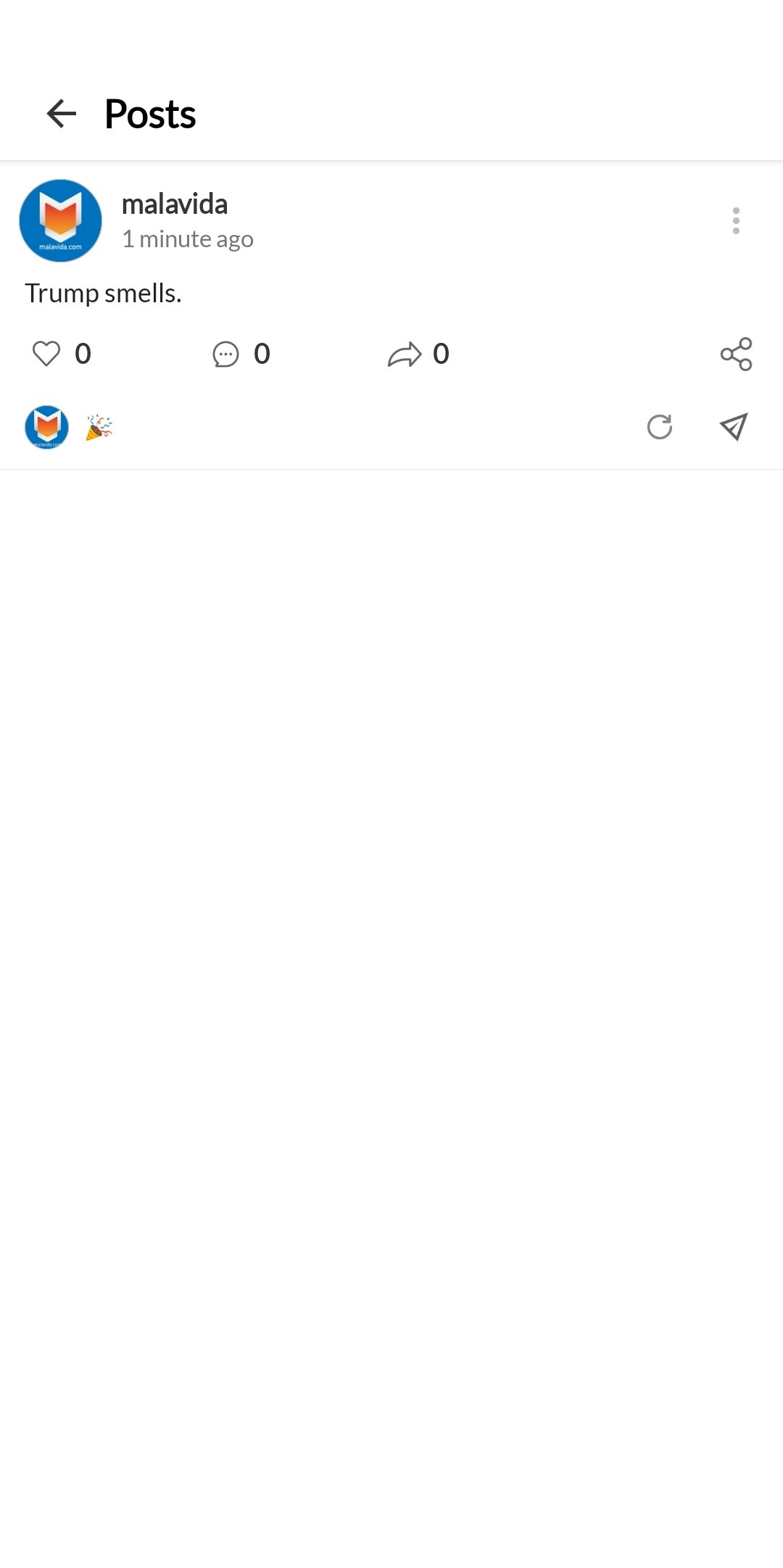The image features a social media post with a predominantly white background. 

- **Top-Left Corner**: "POSTS" is written in black text accompanied by a black leftward-pointing arrow. 
- A fine gray line runs horizontally from the left edge to the right edge of the image.
  
- **Post Header**: Below the gray line, the username "Malavida" is displayed in small black letters, immediately followed by "one minute ago" in gray font. A distinct blue circle with a white 'M' filled in with orange is positioned to the left of the username.

- **Post Content**: The user "Malavida" has posted the text "Trump smells." 

- **Interactivity Icons**: 
  - To the right of the post, there are three vertically aligned gray dots indicating more options.
  - Below the text, there is a series of interactive icons:
    - A gray outline of a heart followed by a '0' in black.
    - A gray chat bubble with three dots and a '0' in black.
    - A gray share arrow with a '0' in black.
  
- **Footer**: 
  - The text "Malavida.com" appears at the bottom.
  - The same blue circle with the white 'M' in orange reappears next to a celebration emoji.
  - To the right, there's a gray circular outline with an upward-pointing triangle, followed by another fine gray line running horizontally across the image.